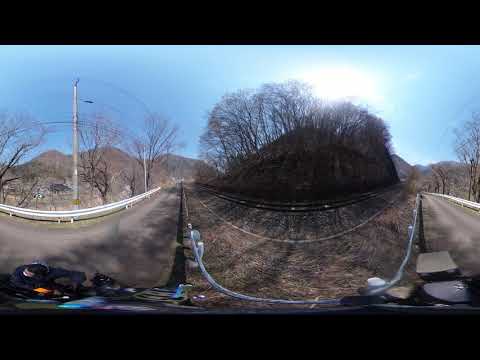This panoramic image shows a curved road bordered with safety barriers and flanked by leafless trees, appearing to split and loop back in the distance. The road starts at the bottom left corner and curves gently, creating a sense of depth as it stretches toward the horizon. A hill with sparse vegetation and trees separates the two lanes, while metal silver barriers line both sides of the road. The bright blue sky and the brilliant sun, positioned behind the treetops on the right, bathe the scene in natural light. There is a telephone pole visible on the left side along with additional light posts dotting the road. In the foreground, a motorbike's speedometer is just visible, indicating the perspective is from a moving vehicle. The narrow two-lane road, devoid of other cars and road markings, gives a tranquil and open feel to the image.